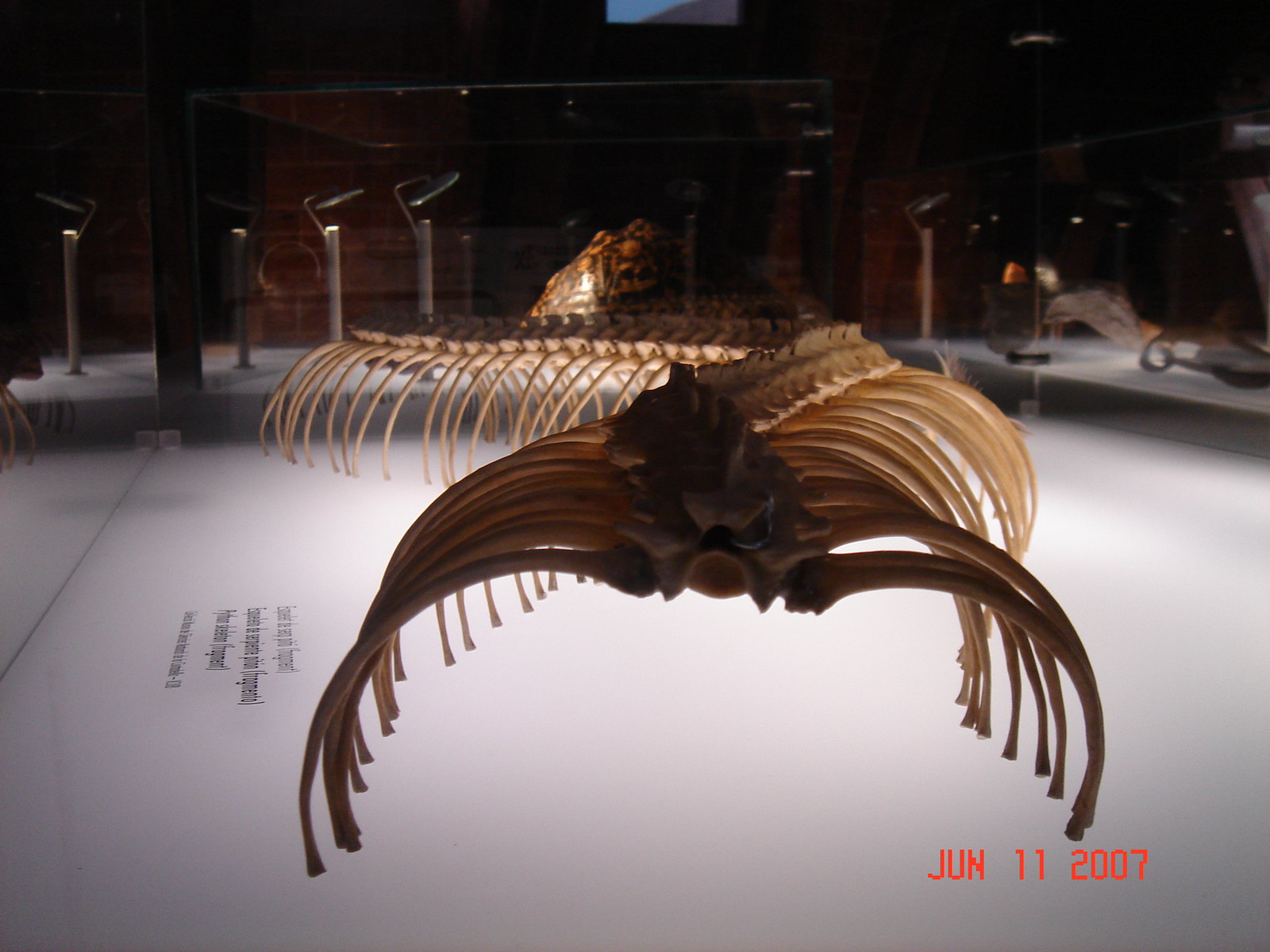This photograph captures a museum exhibit showcasing the skeletal remains of a large reptile, likely a snake, displayed prominently on a white surface that resembles a table or flooring. The exhibit is framed by a rope barrier supported by stanchions, emphasizing its importance and delicate nature. The skeleton's spine curves elegantly in a serpentine S-shape, with dozens of yellowed ribs extending outward, creating an intricate and captivating pattern. The exhibit area is partially illuminated, casting intriguing shadows under the skeleton while the background remains dark, accentuating the exhibit's details. A red timestamp in the lower right corner of the photograph reads June 11, 2007, marking the date the image was taken. Additionally, there is black text on the white floor near the exhibit, likely providing information about the skeletal remains, though it's illegible from the photo's perspective. In the background, fluorescent lights and other exhibit elements are faintly visible, contributing to the overall mysterious and solemn ambiance of the museum setting.